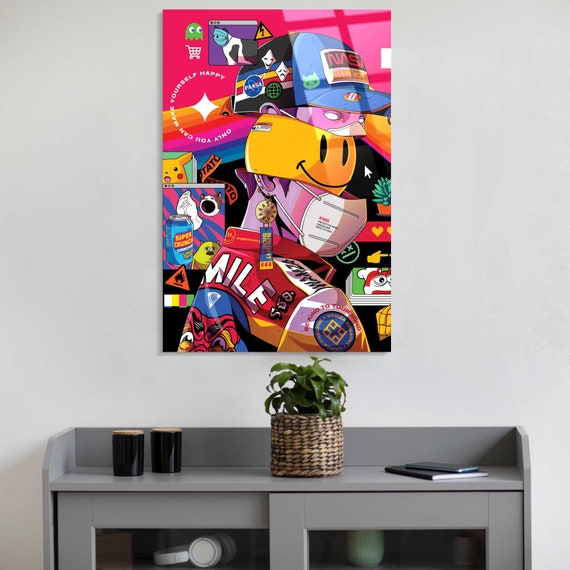The image captures a vibrant and colorful scene inside a room. Dominating the gray wall is a visually striking poster or canvas print in a vertical, rectangular format. The poster showcases a myriad of colors—reds, oranges, whites, blues, essentially the entire spectrum of the rainbow—and features a central theme of a playful, cartoonish blend of a smiley face and the character Pac-Man, with an anime-style face that integrates Pac-Man into its design. This whimsical artwork is adorned with various trinkets and elements, creating a busy yet captivating composition, including a hat that contributes to its lively appearance.

Below this vivid poster, there is a person wearing a white N95 mask and a multicolored jacket with the word "smile" on the back, aligning with the cheerful theme above. Underneath the person's image, a gray cabinet with glass-paneled sliding doors sits against the wall. On top of this cabinet rests a wicker basket containing a small, vibrant green plant, flanked by two black cylinders (likely candles) on the left side and two stacked notebooks on the right. Peeking through the glass doors, you can spot a headset on the left and a green cup on the right, adding to the eclectic assortment of items that decorate this cozy and visually stimulating space.